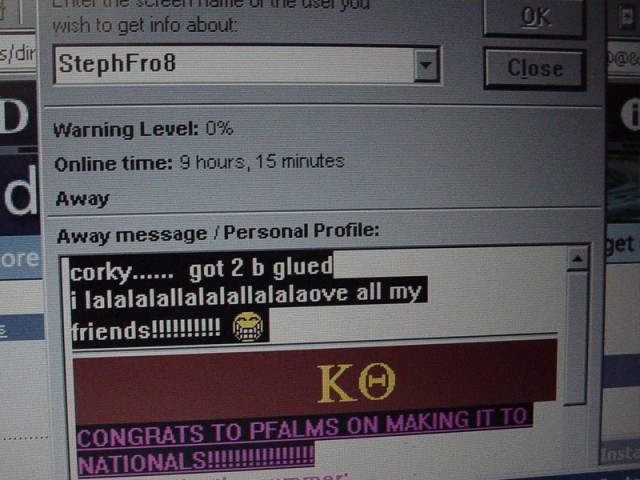The image displays a pop-up dialog box from a Windows computer that resembles the old Windows 95 style. In the gray message box at the top, "StephPro8" is typed in a dropdown tab with an arrow, next to which there are "OK" and "Close" buttons. Below this, in black print on a gray background, it reads: "Warning level: 0%, Online time: 9 hours, 15 minutes," followed by the word "Away." There is a horizontal border, below which it says "Away message / Personal profile." The personal profile section features the text: "Quirky... got to be glued... I la la la la la love all my friends," accompanied by a toothy smiling emoji. Underneath, a maroon banner with gold text reads "KO," with a dumbbell inside the "O." Beneath this banner, on a black background with magenta text, it says: "Congrats to PFALMS on making it to nationals!!!"